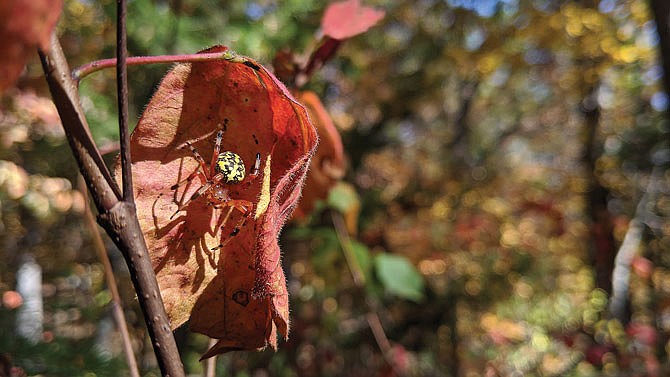In this picture taken outside in a garden, the main focus is a colorful spider prominently perched on a wrinkled reddish-brown and splotched leaf on the left side of the image. The spider, with its elaborate, brilliantly red legs, features a large, striking abdomen that combines black, bright orange, and vivid yellow, making it stand out against the leaf and appear camouflaged on the red flower. The leaf is still connected to a twig that runs from the bottom left to the upper left of the photograph, which is also intertwined with branches. The background on the right side of the image is blurred but filled with patches of vibrant yellow, red, green, and blue hues, suggesting other plants and flowers illuminated by warm sunlight. This blurring emphasizes the spider and leaf as the focal points of the photograph.